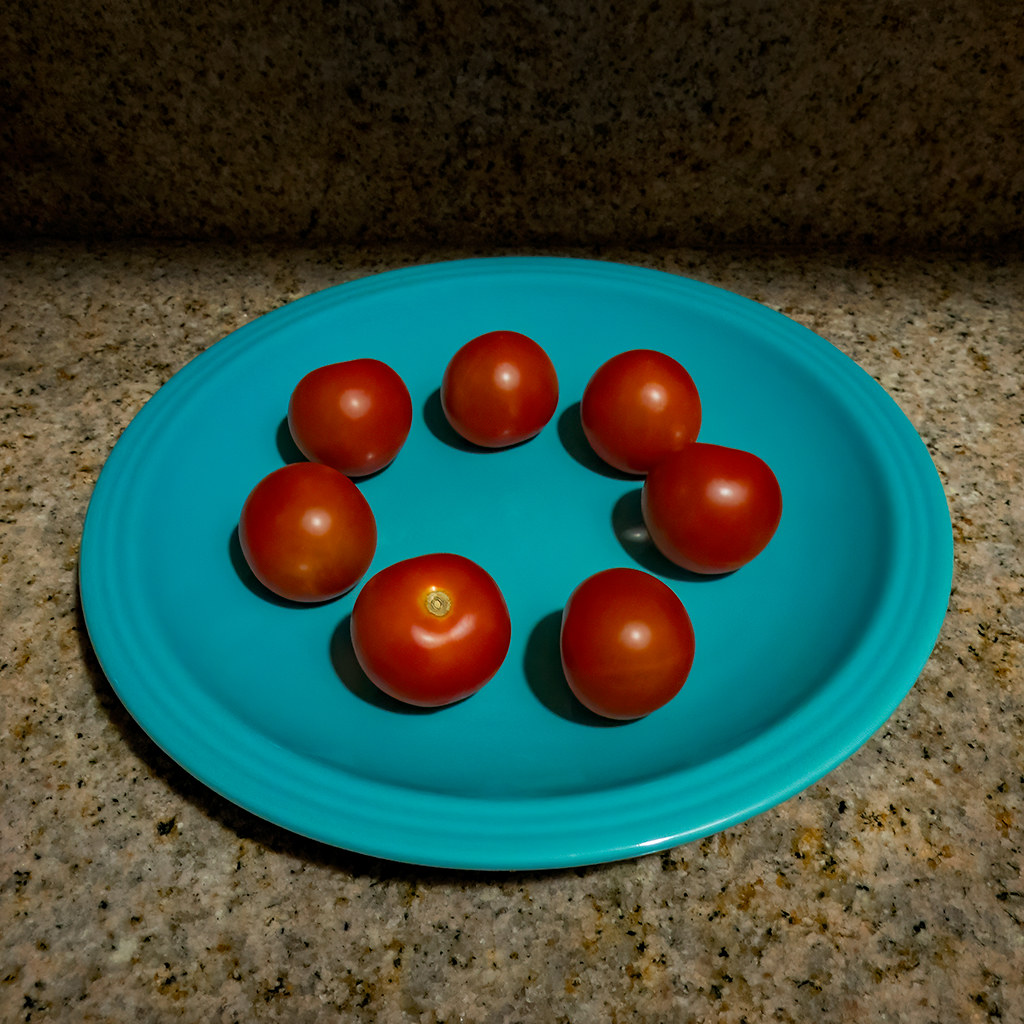This photograph captures an arrangement of seven ripe, bright red cherry tomatoes placed in a perfect circle on a turquoise plate, which appears to be slightly shiny, possibly made of plastic. The tomatoes are positioned on a chocolate brown granite countertop with flecks of black, tan, and gray. The countertop extends into a matching granite backsplash in the background. The light source, likely fluorescent, is coming from the upper right corner of the image, casting sharp shadows and creating small white reflective marks on the tomatoes. The tomatoes vary slightly in size and all but one are facing down, with the single upward-facing tomato displaying a small circular green spot where the stem used to be. The plate also features a ridged edge, adding texture to the composition. The photograph is taken from an angle of about 45 degrees above the scene, highlighting the intricate details of the tomatoes' reflections and shadows.